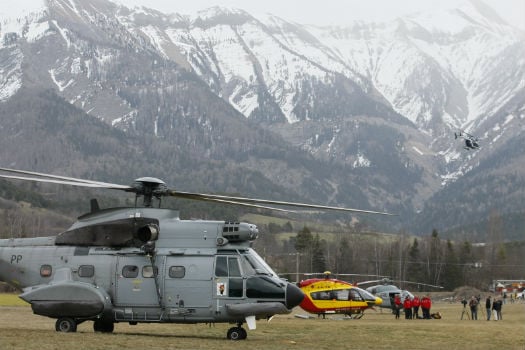The image features three helicopters set against the striking backdrop of a towering, snow-covered mountain. The mountain dominates the background, with its white snowy peaks giving way to darker rock and earth tones lower down. At the base of the mountain, a field populated with green grass and lined with trees serves as the landing area for the helicopters. 

In the foreground, a large, gray and black-nosed transport helicopter is prominently visible. Behind it stands a smaller, vibrant red and yellow helicopter. Further back still, a third, smaller gray helicopter can be seen in the distance.

Centered between the first two helicopters is a group of people. Most of them are wearing red coats and black pants, consistent with the attire of team members or personnel. Among them, a crew is setting up and filming with cameras on tripods, capturing the scene. The presence of the camera equipment and the coordinated outfits of the individuals suggest a professional or organized event, adding a dynamic human element to this outdoor setting. In summary, the image is a harmonious composition of aviation and nature, framed by human activity and the majestic, snow-capped mountain backdrop.